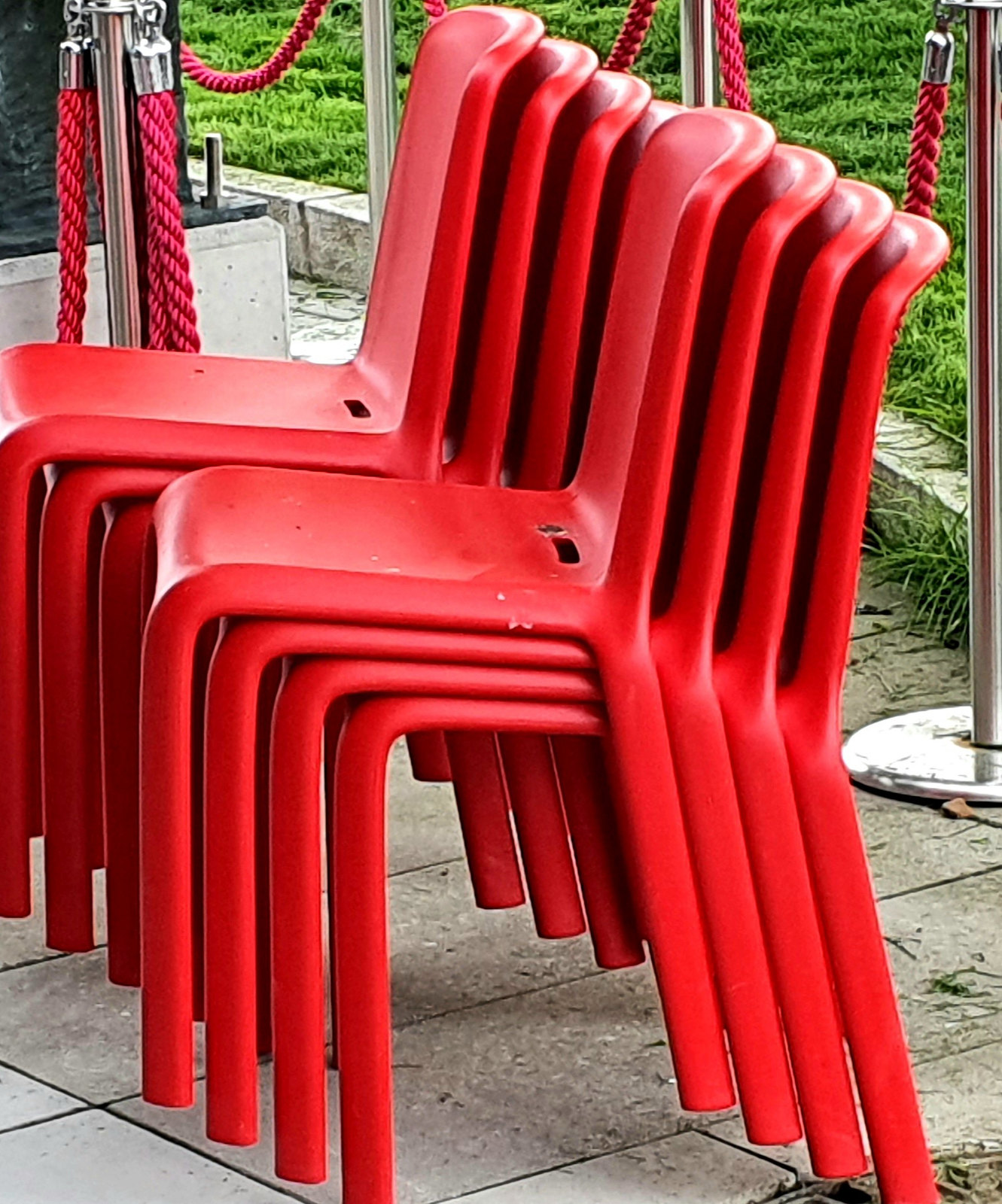The photograph depicts an outdoor scene featuring two stacks of identical red plastic chairs, each stack containing four chairs. The chairs, all without armrests, are prominently displayed in the center of a stone patio area that appears slightly sunken from the surrounding grassy terrain, suggesting a park setting. Rope dividers on metal stands are visible behind the chairs, creating a sense of a cordoned-off space. The stone patio is somewhat unkempt, with grass sprouting through the cracks and around its edges, indicating it hasn't been maintained recently. The overall ambiance is casual and unpolished, with the bulk of the image's focus on the stacked red chairs.